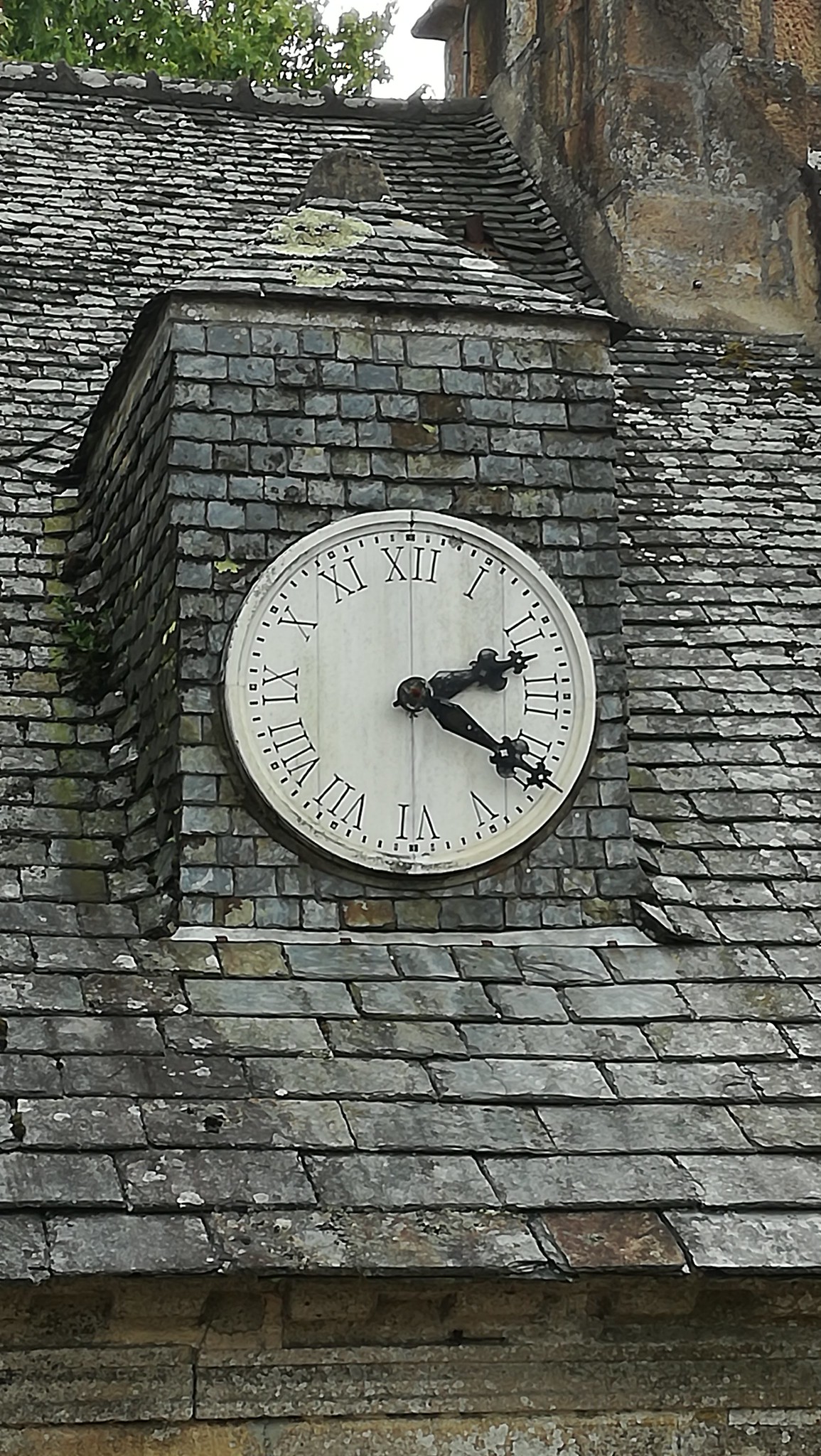The photograph captures a detailed, close-up view of an old, weathered rooftop with dark gray shingles that are slanted and extend from one side to the other. A prominent feature of the roof is a gray stone clock tower that protrudes from the structure. The clock tower, constructed from the same gray stone as the roof tiles, has a large, round white face without any protective glass, exposing the black decorative hour and minute hands and Roman numerals to the elements. The time displayed on the clock reads approximately 2:20. A portion of a differently colored building, likely part of a chimney, is visible in dark stone at the upper right of the image. The background includes some trees visible over the rooftop, and the sky is light in color, almost white. The overall impression is of an older, possibly European, structure with a distinct historical charm. The photograph is taller than it is wide, emphasizing the height and details of the clock tower and roof.